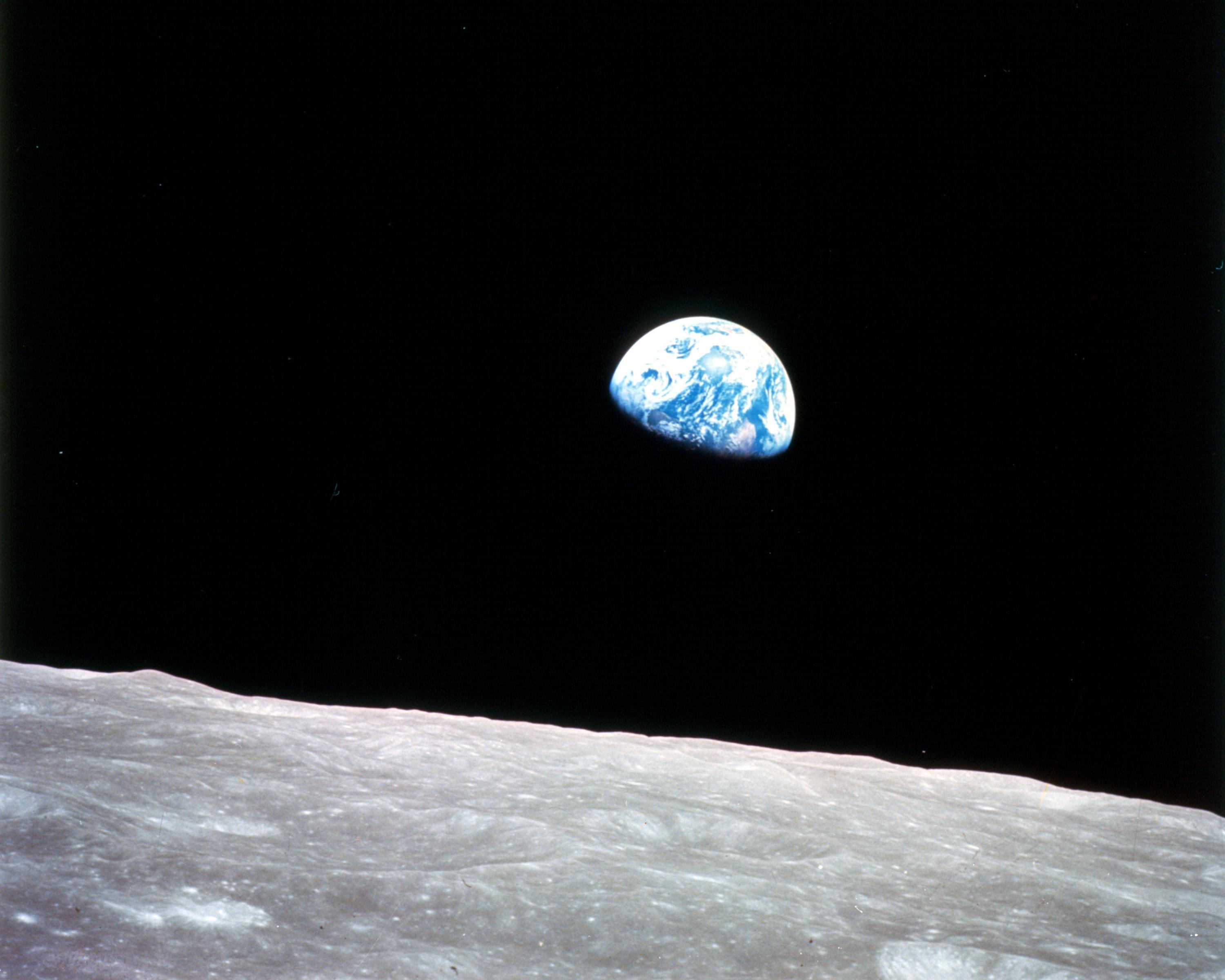In this iconic landscape-oriented image taken from the moon, the bottom third or so depicts a gray, cratered lunar surface devoid of any visible life. Above this stark expanse, the infinite blackness of outer space stretches out, punctuated only by a few faint, distant stars. Dominating the center of the image is the Earth, half-lit by the sun, revealing a breathtaking view of swirling white clouds and sprawling blue oceans. The scene is a striking blend of black, gray, white, and blue, capturing the serene yet powerful presence of Earth suspended in the vastness of space.